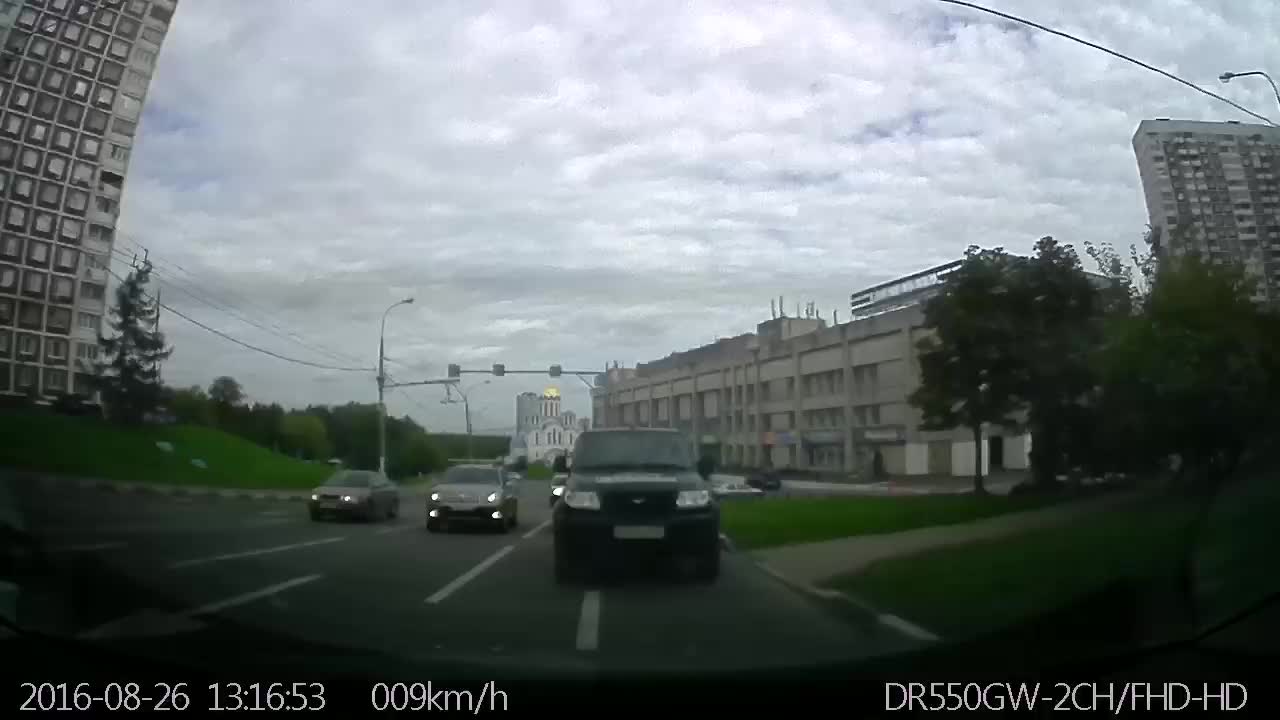Captured from the perspective of a vehicle in motion, this photograph offers a unique rearward view of a bustling four-lane highway. The shot, almost panoramic in appearance due to its rounded edges, encapsulates a stretch of road bordered by two curved buildings that frame the scene. The sky above is densely clouded, casting a muted light over the surroundings. In the distance, a mix of buildings, trees, and grassy hills provide a varied backdrop.

Multiple vehicles trail the photographer's car, the closest being a dark truck or SUV without its headlights on. Surrounding this vehicle are several smaller cars, all with their headlights illuminated, likely as a safety measure under the overcast skies. 

A digital time stamp that reads "2016/08/26 13:16:53" is visible on the image, indicating the date and precise time the photo was taken. Additionally, the notation "009 kilometers per hour" suggests the current speed of the photographer’s vehicle. Off to the right side of the image, in capital letters, the model of the recording device is indicated as "DR550GW-2CH-FHD-HD," further attesting to the detailed metadata captured along with the photograph.